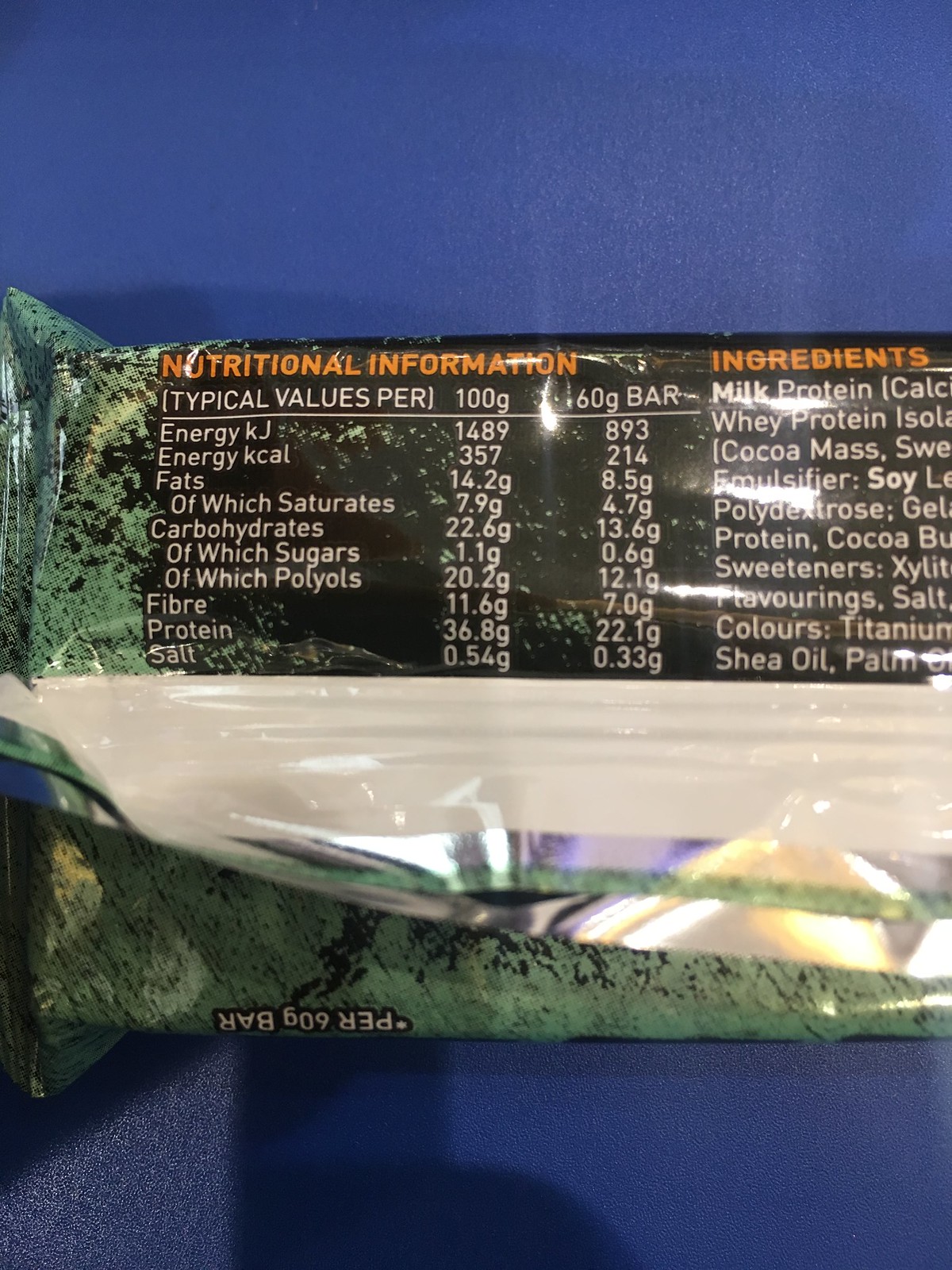A detailed view of the back of a protein bar’s packaging. The image is vertically oriented, though the bar itself is placed horizontally and only the left side is visible. The background features a gradient blue, transitioning from a medium blue at the top to a darker hue at the bottom due to shadowing. The wrapper of the bar displays a lighter green background with gray or black splotches. The focal point is the nutritional information section, which has a black background with orange text. Beneath this, white text lists the typical values per 100 grams and per 60 grams bar, including energy in kJ (1489 and 893 respectively), energy in kCal, fats, saturates, carbohydrates, sugars, polyols, fiber, protein, and salt. Ingredients are partially visible, listing milk protein, whey protein, cocoa mass, emulsifier, soy, sweeteners, and shea oil among others. The lower part of the packaging is folded down, revealing a white strip and more of the light green background.